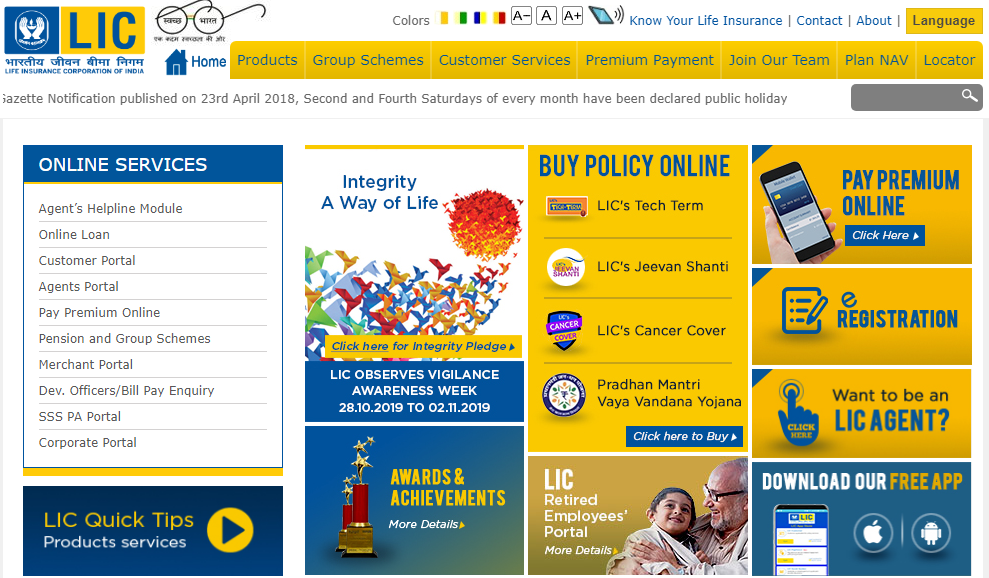**Caption:**

In the upper left corner, there is a blue box beside a yellow box containing the letters "L-I-C." To the right, there is an image of a small pair of eyeglasses. Below this, a house symbol appears beside the word "Home." Inside a long yellow box are the following options: Products, Group Schemes, Customer Services, Premium Payment, Join Our Team, Plan NAV, and Locator. A gray box contains the text "Lisette notification published on 23rd April 2018. Second and fourth Saturdays of every month have been declared public holidays." To the right, another gray box displays a magnifying glass symbol. On the next row, a blue box labeled "Online Services" is followed by choices: Online Loan, Customer Portal, Pay Premium Online, and Corporate Portal. Over to the right, there are different boxes; one yellow box offers the option "Buy Policy Online." Below this, an image depicts a man with glasses smiling with a young child on his lap, captioned "L-I-C Retired Employees Portal." To the right, an image of a cellphone is accompanied by the option "Pay Premium Online" with a "Click Here" prompt. Below that, an image of a notebook appears beside the word "Registration."